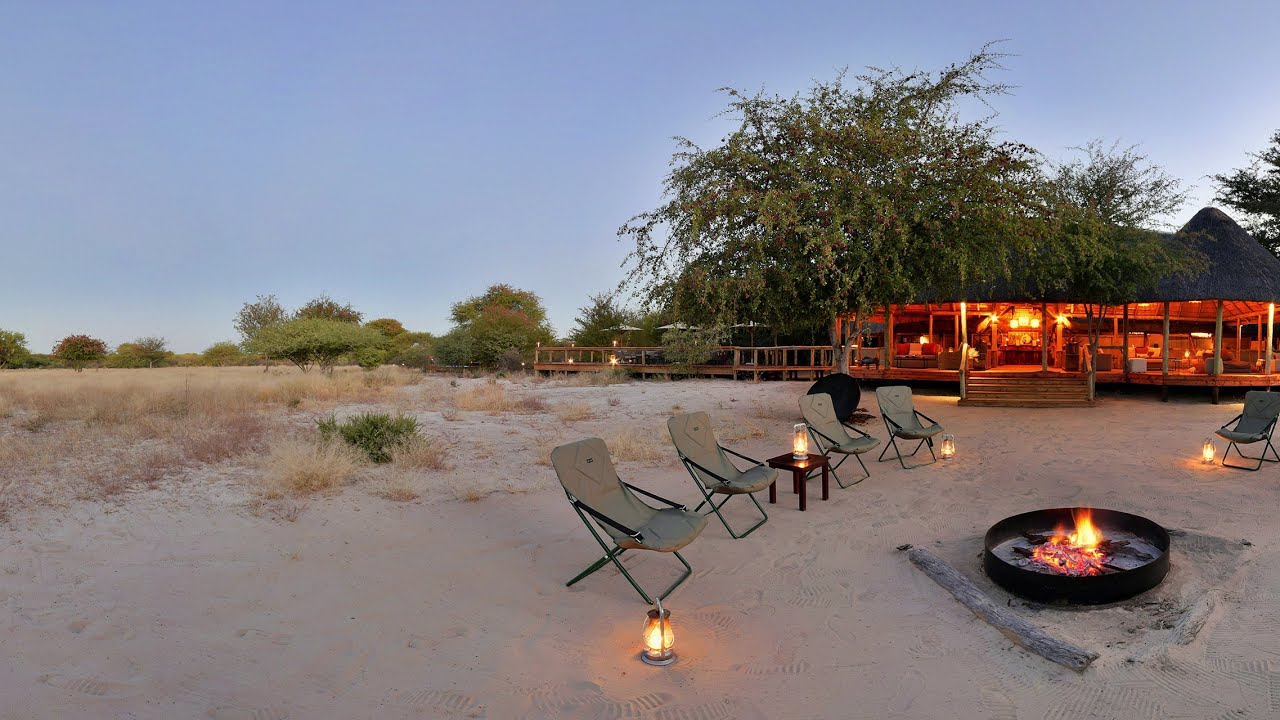This horizontal rectangular photograph captures a serene beach scene at dusk, featuring a well-set campsite. In the foreground, four substantial beach chairs are positioned in a semi-circle around a circular fire pit with a lively fire. An additional chair is located to the right, partially cut off by the frame. Small lanterns are scattered around the chairs, with one resting on a wooden side table between two of the seats, enhancing the ambient light. The sandy area with sparse dry grass and green shrubs suggests a coastal environment, possibly a beach. In the background, a well-lit, red-hued wooden pavilion with an open front and a roof is visible, likely a beach house or a restaurant. The structure is flanked by trees, and the clear blue sky above completes the tranquil outdoor setting, indicating preparations for a charming evening by the sea.